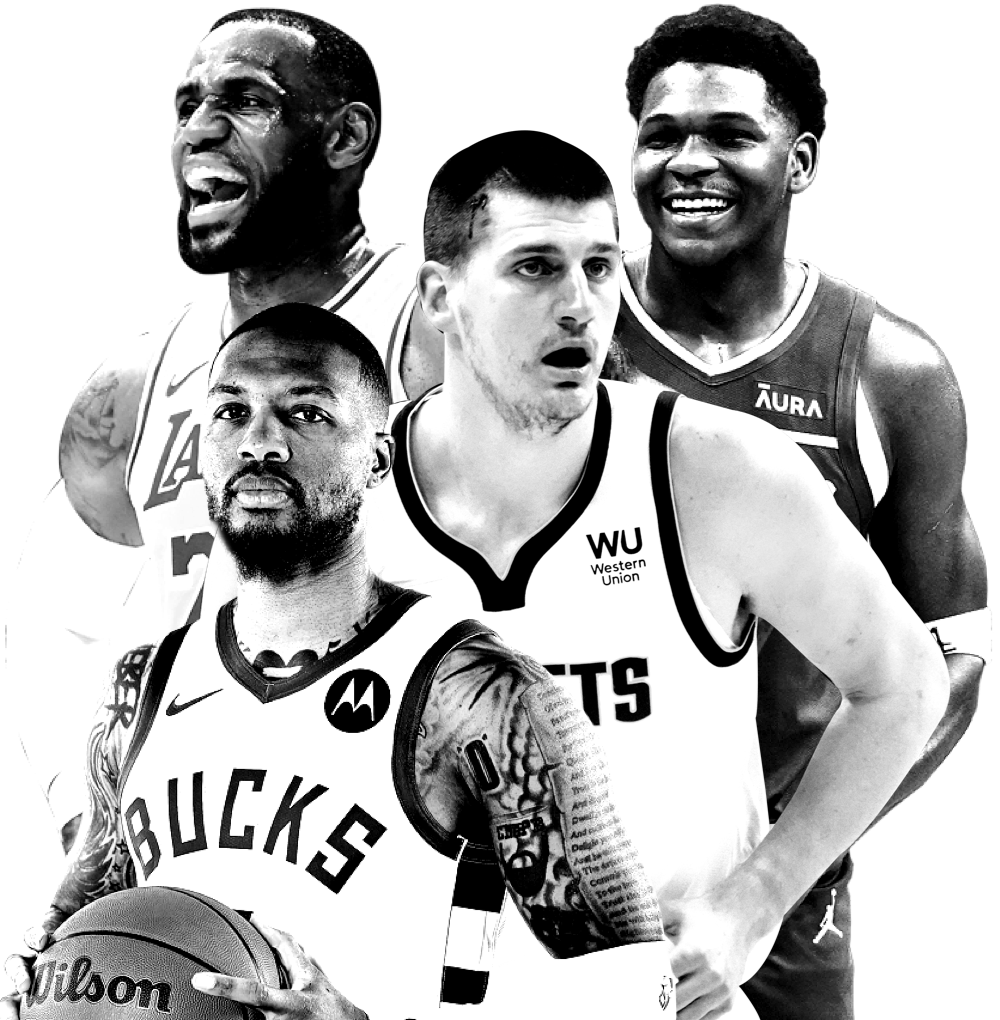This black and white photograph showcases four NBA players in a striking promotional image against a plain white background, suggesting it was taken either in front of a green screen or expertly edited to have no background distractions. Prominent in the image are modern brands such as Nike, Motorola, Western Union, and Wilson, indicating it is contemporary. On the top left, LeBron James is captured with his mouth open, face turned to the left, showing some perspiration. He is sporting a Lakers jersey with the Nike swoosh visible on the right chest area. Below him is Damian Lillard in a Milwaukee Bucks jersey, holding a Wilson basketball with both hands; the Motorola logo is evident on the left chest of his jersey, and his arms are covered in tattoos. Behind Lillard, another player wears a jersey marked with the Western Union logo on the left chest. To the right of him, another player smiles broadly, revealing all his teeth. This image, intensely focused on the players, appears to be a modern promotional poster or advertisement, given the emphasis on current team logos and branding.